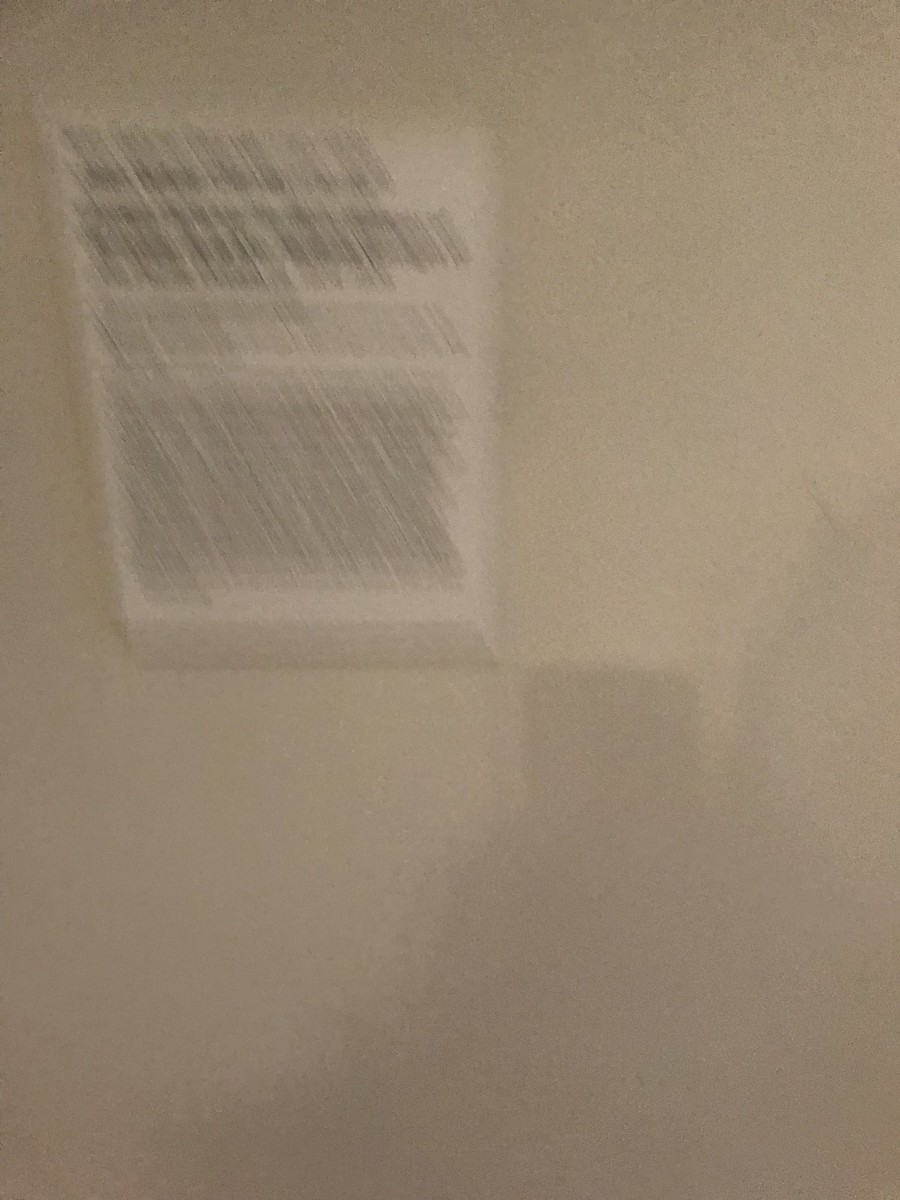A blurry photograph captures a white wall with a piece of paper affixed to it. The paper, also white, contains four paragraphs of text. The first two paragraphs are bolded and written in black ink. In contrast, the third and fourth paragraphs are not bolded, with the fourth paragraph being particularly lengthy. Due to the blurriness of the image, the text on the paper is indistinguishable. Additionally, a shadow on the bottom right side of the image appears to show the top of a person's head and the edge of a cell phone, suggesting someone is holding the phone up to take the picture. The photo appears to be out of focus and does not seem to have any filter applied.